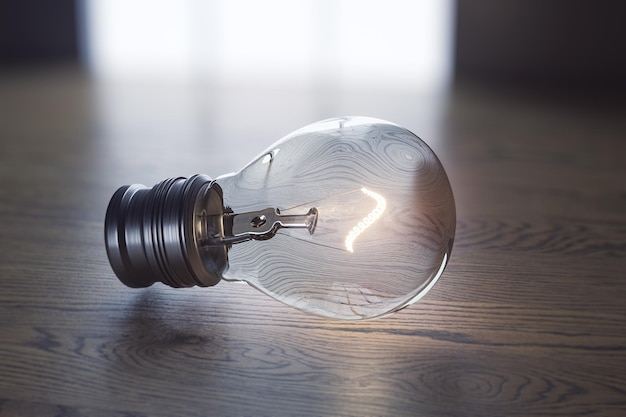This detailed image features a vintage-style decorative light bulb appearing to levitate slightly above a dark wood grain floor or desk with a blurred, light-filled window in the background. The ornate bulb, which has a glass exterior and a brass or copper-colored base, is illuminated from within. Through the clear, thick glass, which distorts the wood grain beneath, the filament can be seen glowing with an orange hue, despite the lack of a visible power source. This filament forms a thick, S-shaped pattern resembling the inner workings of an antique lighter. The overall atmosphere of the image suggests a digitally altered or AI-generated scene, enhancing the antique and decorative aesthetic of the bulb.